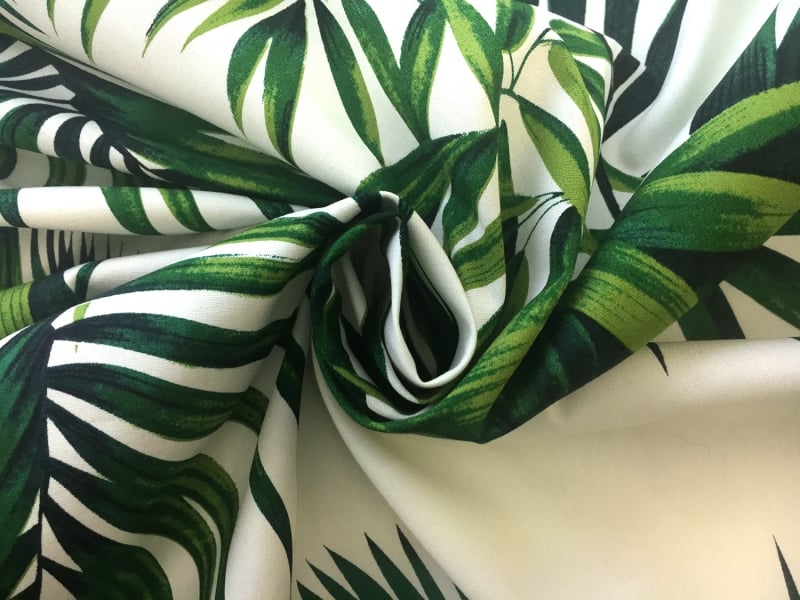A detailed observation reveals an intricately designed cloth, predominantly featuring a blend of white and green hues. The cloth seems to be bunched up in the middle, somewhat twisted, giving an impression of a blooming flower. The design showcases an array of sharp, thin leaves, varying in shades of green, interspersed with white spaces. The upper right section prominently displays a dense green leaf pattern while the rest of the cloth alternates between green leaves and white spaces. Light illuminates the upper part of the cloth, casting a shadowed effect towards the bottom right. The texture indicates a fabric-like material, possibly a tablecloth, although its exact nature is indeterminate due to the crumpled state. No additional objects or text are present in the image, keeping the focus solely on the ornamental leaf motifs and the interplay of light and shadow on the bundled fabric.